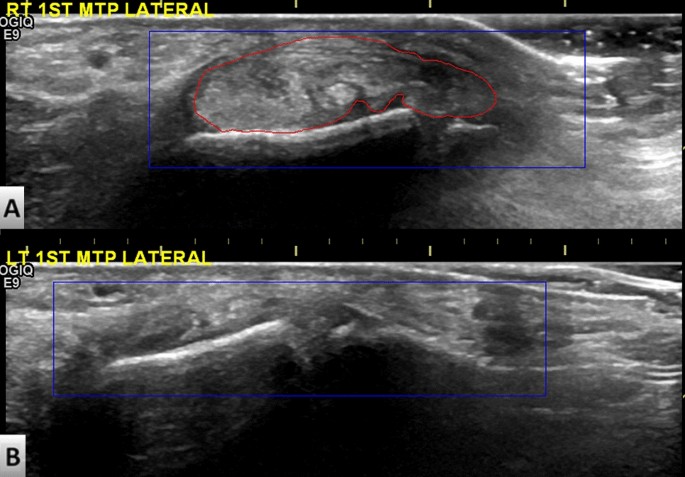The image consists of two stacked ultrasound scans of metatarsophalangeal (MTP) joints, labeled as "RT, 1ST, MTP lateral" in the top image and "LT, 1ST, MTP lateral" in the bottom image. Both images, displayed on a black background with shades of gray and occasional haziness, are surrounded by blue rectangles highlighting focal points within the joints. The top image additionally features a red curved line emphasizing a specific area, whereas this detail is absent in the bottom image. Text in the upper section of both images includes the code "OG1QE9." The scans depict the joints with a focus on potential abnormalities such as deformation or degradation, particularly visible in the top-right MTP joint. These structural evaluations of the metatarsophalangeal joints suggest a clinical examination, possibly to diagnose or monitor joint health issues.